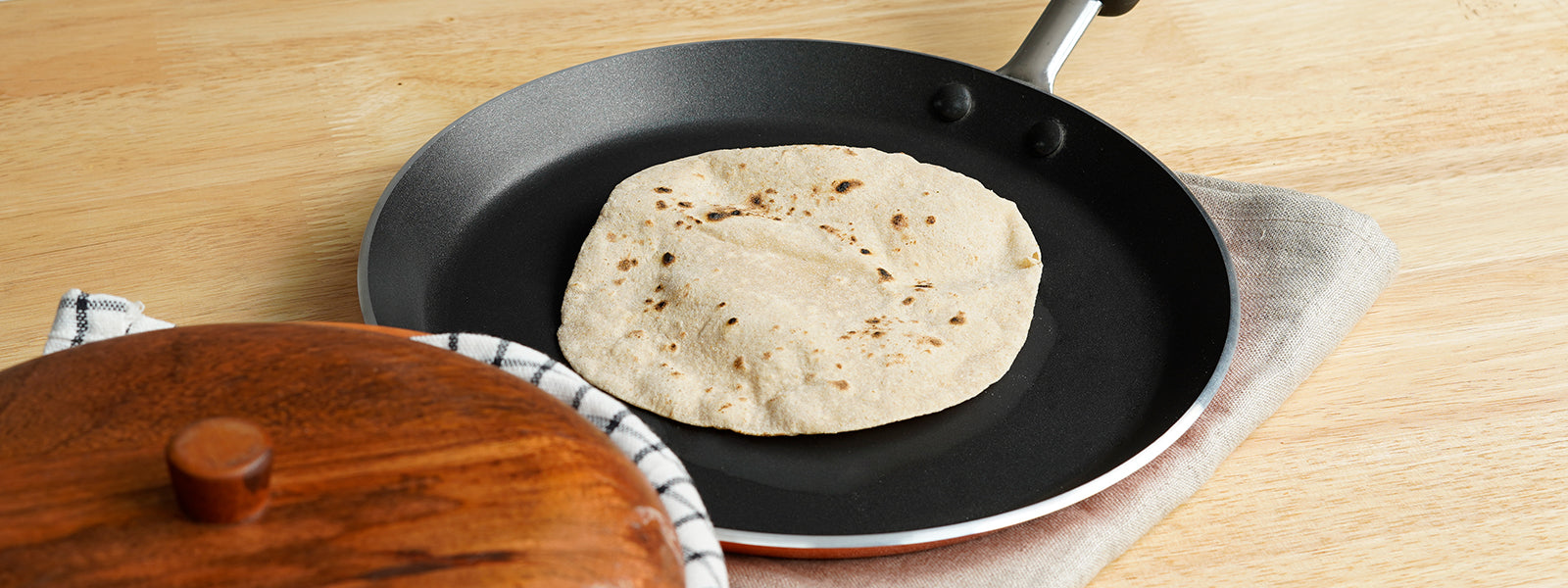The image captures a black non-stick skillet centered on a white folded towel, which rests on a wooden surface showcasing its visible grain. Inside the skillet, a flour tortilla with dark brown speckles is cooking. Diagonally to the lower right corner, there is a dark wooden tortilla serving dish with a lid, which holds a towel featuring thin blue stripes. The skillet's silver handle and the contrast between the black interior and the white tortilla form a striking visual focus. The overall composition of the image is a horizontally long rectangle, emphasizing the central placement of the skillet.